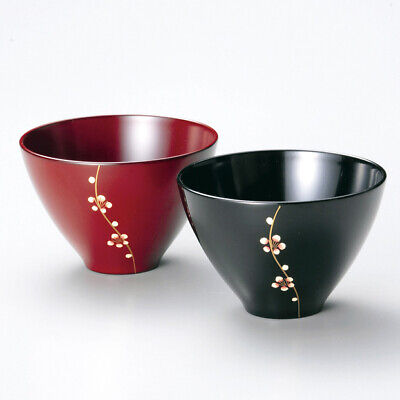This image features two elegant bowls set against a light gray background. Each bowl, tapering from a wider opening to a narrower base, radiates an oriental aesthetic. The bowl on the right is a glistening black with a reflective interior, while the one on the left exhibits a rich amber red hue. Both bowls are adorned with intricate, vine-like brown stems that wind gracefully from the top to the bottom. Sprouting from these stems are several delicate white buds, each accented with a hint of red at their base, giving a sense of blossoming life. The bowls' surfaces gleam, suggesting a ceramic or metal material, further enhancing their refined appearance.